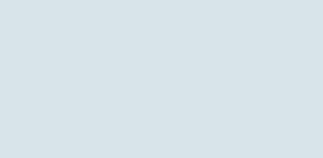The image features a plain, rectangular box colored battleship gray, measuring approximately two inches in height and four and a half inches in length. This nondescript, unadorned box sits adjacent to another section labeled "Think About" which contains various intriguing elements. The "Think About" section suggests examining details such as the image's composition, the relative positions of objects, and the accompanying text. In contrast, the gray box stands out due to its simplicity, lacking any discernible features or subtle details, and blending seamlessly into the battleship gray background. The overall aesthetic is minimalistic, highlighting the absence of objects and imagery within the gray box.